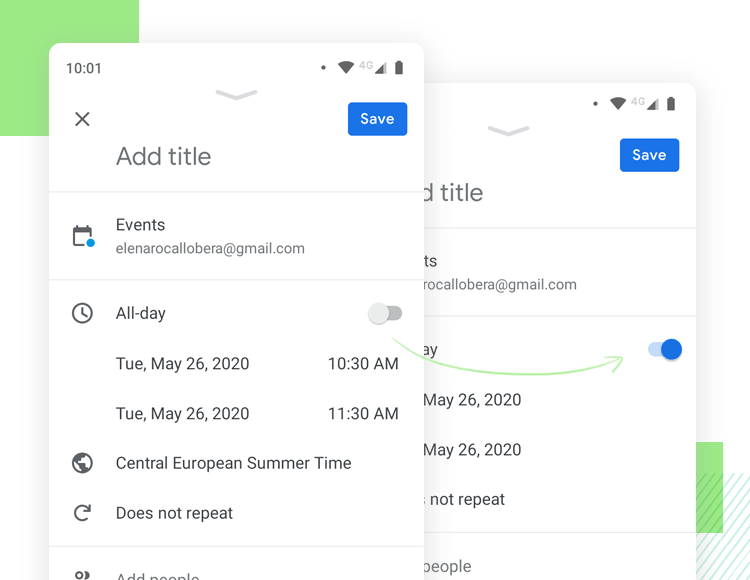Two screenshots display smartphone pages designed for adding titles to calendar events, complete with various interface elements and timestamps. The first screenshot shows details partially obscured by the second screenshot. The visible timestamp on the first screenshot reads 10:01, accompanied by indicators to its right—a black dot, Wi-Fi logo, 4G logo, and battery icon.

In both screenshots, a dropdown arrow appears in the middle of the screen, and beneath it are functions to either close the current screen, save the title, or add a title. Below these functions, a calendar displays linked to the email elainarocolbera@gmail.com. Both screenshots also feature an 'all day' toggle switch associated with a clock icon; in the first screenshot, this feature appears off, whereas in the second, it is switched on, indicated by an arrow showing the change.

Further down, both screenshots show an event scheduled for Tuesday, May 26, 2020—one at 10:30 a.m. and the other at 11:30 a.m. The second screenshot’s details are partially covered, repetitively showing the same date, but only the times 10:30 a.m. and 11:30 a.m. can be seen clearly.

Towards the bottom of the visible screenshot, there is an Earth logo indicating the time zone, marked as Central European Summertime. Adjacent to this is a half-circle refresh button labeled "do not repeat." This "do not repeat" setting and an option to "add people" are consistent across both screenshots.